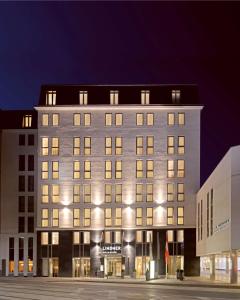The image depicts a detailed 3D architectural elevation of a multi-story building at nighttime, set against a dark blackish-blue sky. The structure, likely a hotel or a residential building, stands prominently with a flattish roof adorned by five dormer windows. The building is composed of light-colored brick from the top, with the bottom two floors featuring a dark brick façade. There are approximately eight stories, including the ground level which features significant glass frontage and a covered section with visible shops. The entrance is marked by four or five columns, with the outer ones painted black and the inner ones gray. Bright floodlights illuminate the base of the building, both pointing up and down. Each floor features a set of double windows, arranged five across, making a total of 30 windows visible, including those in the dormer. The marquee hints at a partial name, possibly "Lindbeg." The building is nestled between two adjacent structures: a grey-colored building with columns on the right, and another darker, less lit building on the left. A small beige-colored courtyard and a section of the roadway are visible in front of the building, emphasizing its urban setting.